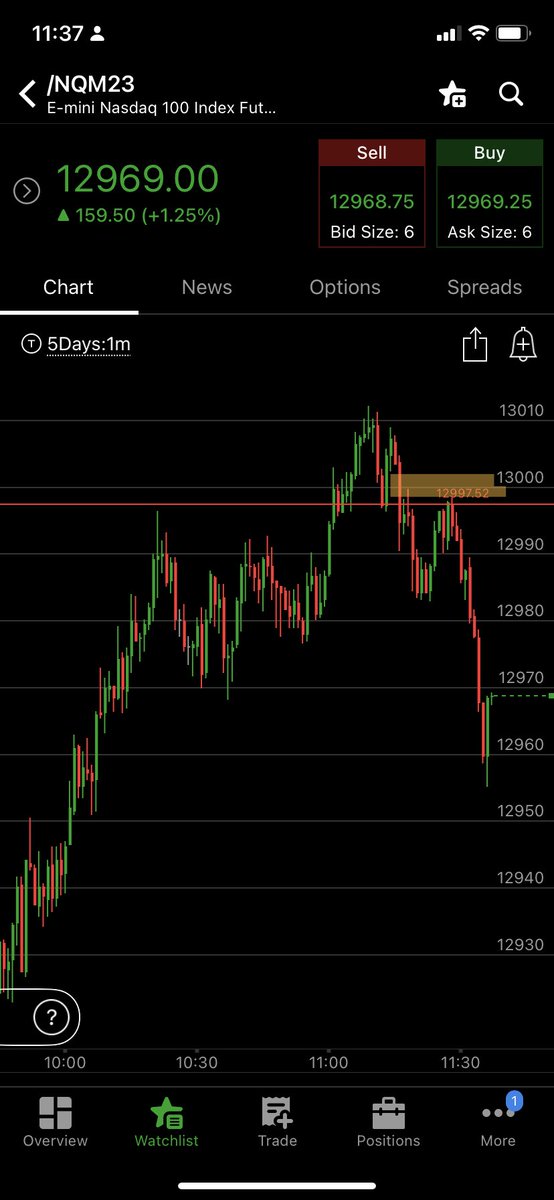This screenshot showcases the A-Stock app interface. In the upper left corner, the current time displayed is 11:37. The upper right corner shows the cell phone reception, Wi-Fi, and battery status icons. Below the status bar, the title reads "NQM23," indicating the specific trading instrument in view. The app further identifies the instrument as the "E-mini NASDAQ 100 Index FUT," followed by ellipses. The main numerical display shows a value of 12,969, presumably in dollars. Beneath this, a green up triangle indicates a positive change, with an increase of $159.50, equating to a 1.25% rise. A graph beneath this information visually represents the performance trend of the E-mini NASDAQ 100 Index over a period.